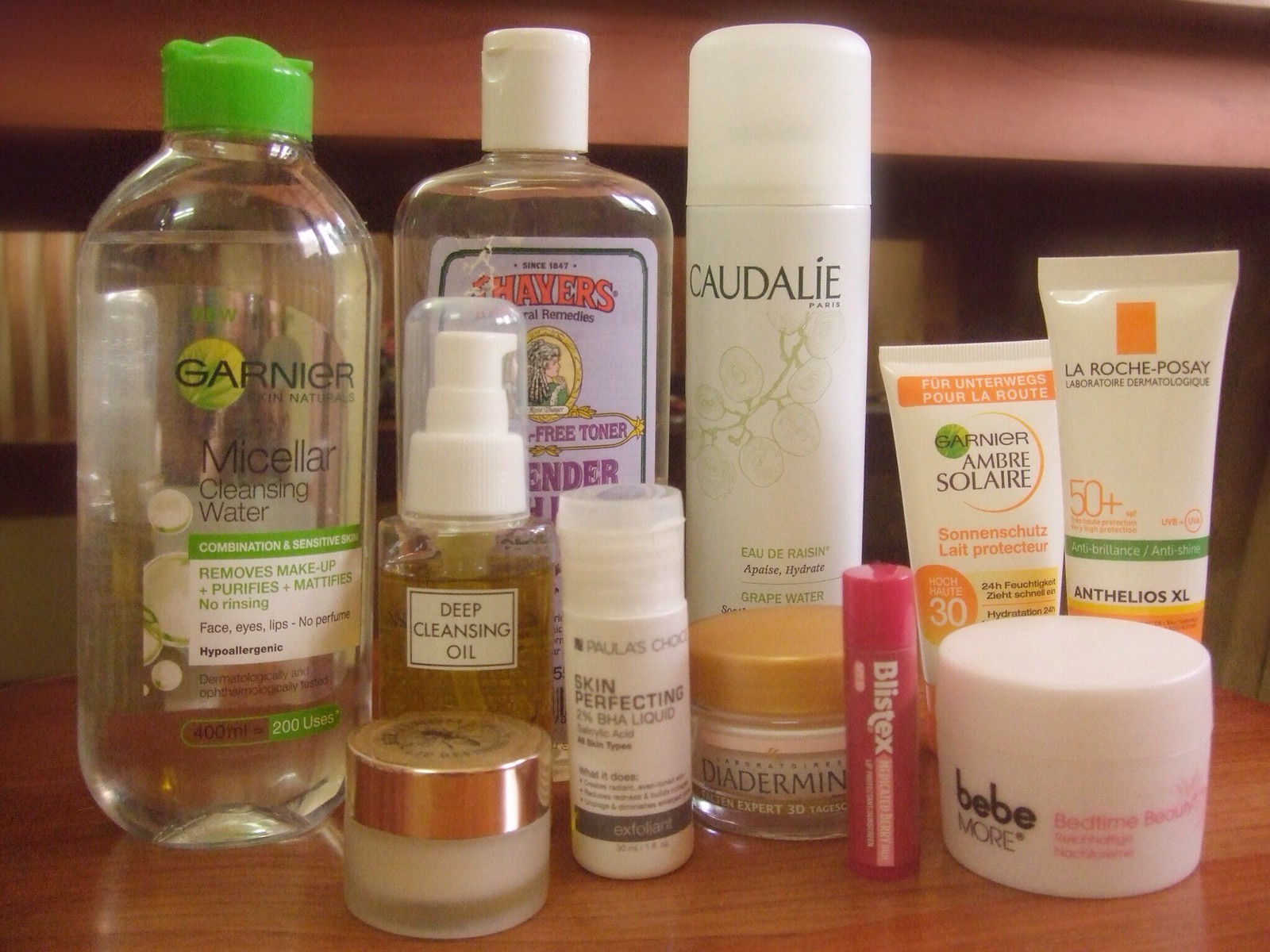The image showcases a reddish-blonde wooden tabletop adorned with various bathroom essentials, including cosmetics, oils, and cleaners. On the far left sits a large, clear bottle labeled "Garnier Micellar Cleansing Water." This bottle features a green cap and a green-and-white label detailing its makeup removal, purification, and moisturizing benefits, which require no rinsing. Positioned just in front of this bottle, slightly to the right, is a small glass container filled with a cream-colored substance, capped with an ornate gold lid featuring a black design.

Directly behind the small glass bottle and adjacent to the Garnier Micellar Water, there is a plastic bottle containing deep cleansing oil. This bottle is equipped with a white pump top secured with a plastic cap. Further to the right and standing behind the deep cleansing oil is a significantly taller clear bottle labeled "Thayers," which appears to contain lavender water. This bottle has a white flip-top cap and features a white label with black and lavender accents.

In front of the Thayers bottle and next to the deep cleansing oil is a smaller white bottle with a clear white flip-top. It has a green band and is labeled as skin perfecting oil. Beside this is another small glass bottle labeled "Datarime," topped with an orange-gold cap.

Behind the Datarime bottle and next to the Thayers bottle is another tall spray bottle marked "Caudalie." This bottle has a white cap, through which a nozzle is visible. In front of the Datarime container stands a pink tube of lipstick, neatly positioned on its edge.

Adjacent to the lipstick tube is a white, round container identified as "Baby Morel," which can be unscrewed to access the cream inside. Behind this setup, there are two tubes of sunscreen: the one on the right is labeled "Garnier Ambre Solaire" SPF 30, and the one next to it is "La Roche-Posay Anthelios XL" SPF 50+.

In total, there are eleven bottles and containers neatly arranged on this wooden countertop.